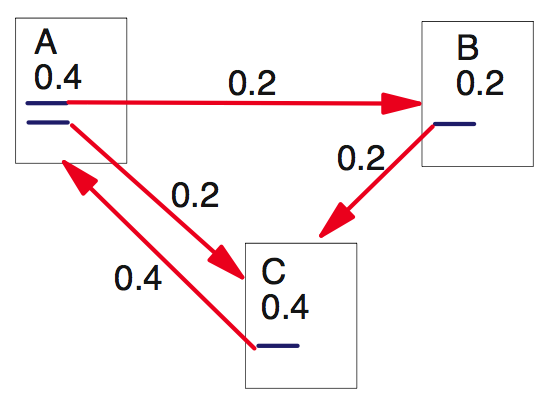This image depicts a schematic diagram illustrating relationships and weight distributions between three labeled boxes: A, B, and C, each with an associated numeric value. 

1. At the top, a white box labeled "A" with black lettering contains the value "0.4." A blue line underlines this box, and there is a distinctive red arrow originating from this box.
2. The red arrow, partially labeled with "0.2," points diagonally downward to the right towards a white box labeled "B" with the value "0.2." This "B" box also features a blue underline.
3. Another blue arrow extends from "A" to a white box labeled "C" with the value "0.4," also containing a blue underline and positioned diagonally downward to the left of box "A."
4. Additionally, an arrow from "C" directs upwards back to the "A" box, indicating a reciprocal relationship. 
5. Lastly, a short arrow from the "B" box points downward to the "C" box, completing the configuration.

The boxes are prominently displayed in a minimalistic color palette primarily comprising white and black, with the red arrow offering a vivid contrast that draws attention within the otherwise restrained graphic.